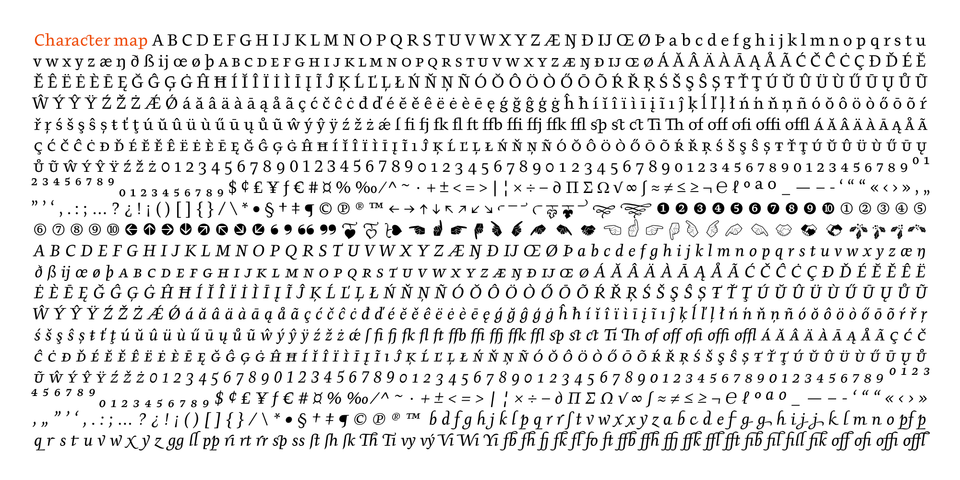Caption: 

A detailed screenshot of a program's font selection interface labeled "Character Map" in prominent red text at the upper left corner. The image displays 21 rows, each showcasing the complete alphabet from A to Z in different fonts, providing a comprehensive perspective on the diverse typographic options available. With around 100 distinct fonts presented in neat rows against a stark white background, the black lettering of each font style enhances visibility and contrast, making comparison straightforward. This visual guide is an exhaustive catalog of font choices for users, tailored for easy selection and application within the program.